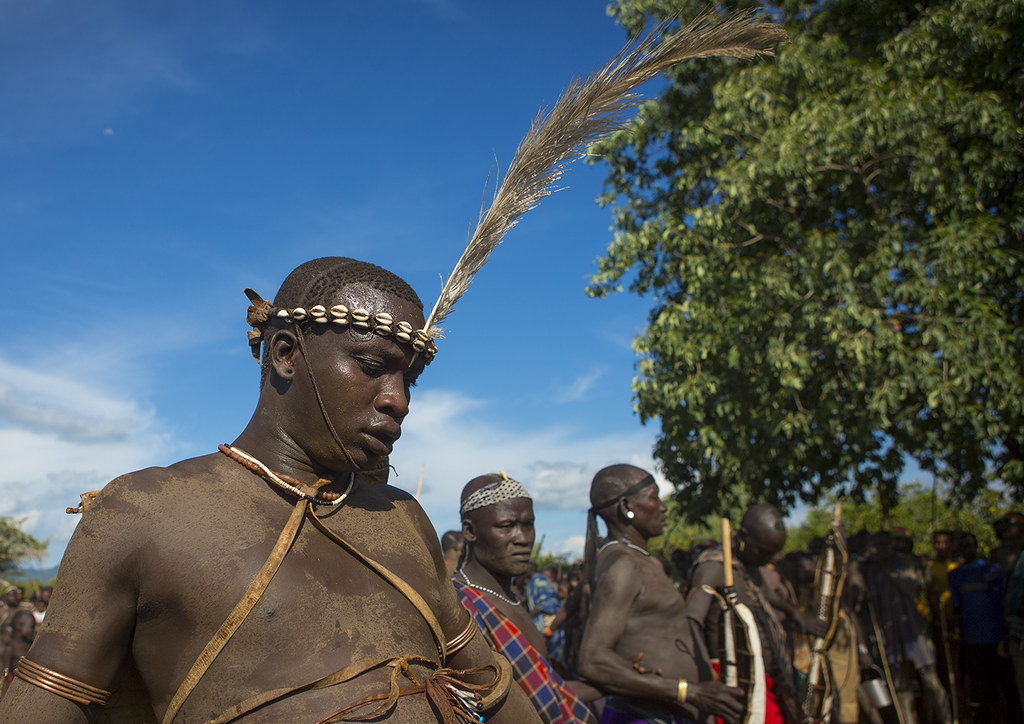The photograph captures an outdoor scene that appears to be in Africa, showcasing a group of tribal men. The sky above is a bright blue with a few white clouds towards the horizon. A large, lush, leafy tree is slightly out of focus in the background on the right side. In the foreground, several dark-skinned, shirtless men are adorned in distinctive tribal ceremonial attire. The man at the forefront wears a headband made of bones with a long feather protruding dramatically, along with leather straps across his bare chest and a copper coil around his upper arm. Similar outfits are seen on the men behind him, featuring headdresses or crowns with feathers and seashells, and red and blue toned fabric. These men are likely involved in a tribal ceremony, observed by a clothed crowd in the background, indicating a possible cultural or ritualistic gathering. The atmosphere and setting suggest a jungle environment, with various trees adding to the tropical feel of the scene.